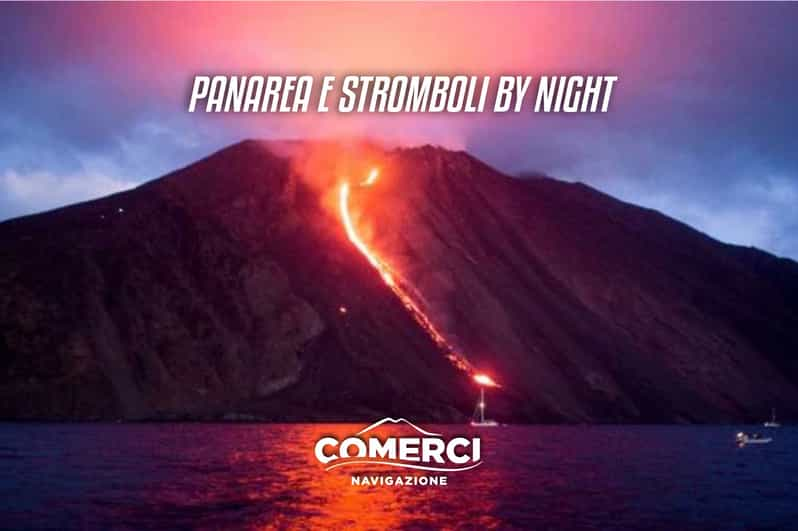The image vividly depicts an erupting volcano by a dark blue body of water. Fiery orange lava cascades dramatically from the volcano's summit, creating a striking reflection in the water below. In the sky above, the eruption illuminates a portion with a vibrant glow, contrasting against the blue, cloud-streaked expanse where the sky remains unaffected. White, italicized letters at the top of the image announce "PANAREA E STROMBOLI BY NIGHT," while the bottom features the text "COMERCI NAVIGAZIONE." In the serene foreground of the reflection-streaked water, at least three boats are visible, one distinctly a sailboat, basking in the glow of the fiery spectacle.